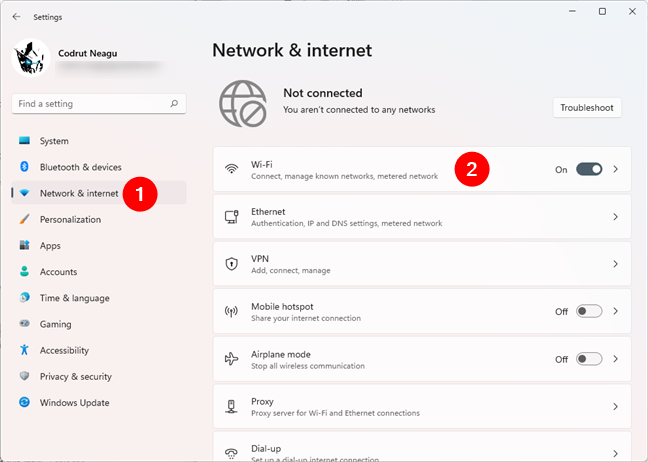Screenshot of the Network and Internet Settings on a Windows PC

This detailed screenshot captures the Network and Internet settings interface of a Windows PC, belonging to the user Kondrut Nigegu, whose profile picture is an anime avatar encased in a white circle.

On the left-side pane of the interface, a comprehensive settings list is presented. At the top of this pane, the user's name is displayed, followed by a 'Find a Setting' search bar. Below this, there are approximately ten listed options, each paired with its respective icon:

1. System
2. Bluetooth & devices
3. Network & internet (highlighted with a red circle containing the number 1)
4. Personalization
5. Apps
6. Accounts
7. Time & language
8. Gaming
9. Accessibility
10. Privacy & security
11. Windows Update

The right-side pane is titled "Network & Internet" and features a globe icon crossed with an 'X', indicating "Not connected - you are not connected to any networks." Towards the far right, a 'Troubleshoot' button is available for potential connection issues. Each section within this pane is organized with a white backdrop, visually separating them.

Each network section consists of an icon, a title, descriptive text, and some sections have toggles for on/off functionality:

1. **Wi-Fi** 
   - Description: "Connect, manage known networks, metered network"
   - Status: Toggled ON
   - Red indicator: 2 notifications

2. **Ethernet**

3. **VPN**
 
4. **Mobile Hotspot**
   - Status: Toggled OFF

5. **Airplane Mode**
   - Status: Toggled OFF

6. **Proxy**

7. **Dial-Up**